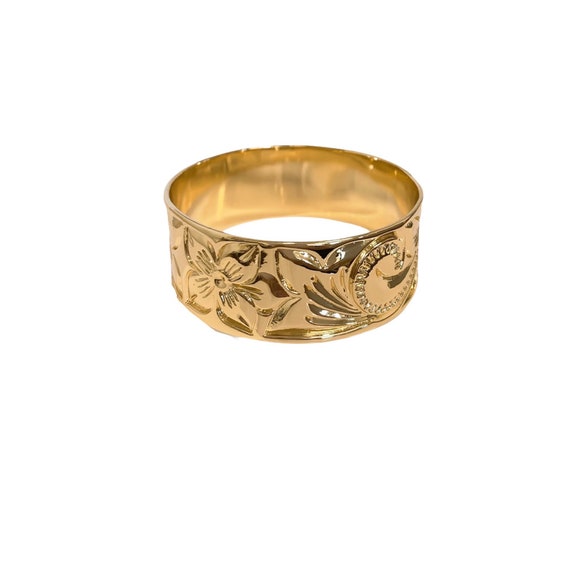This image showcases a close-up of what appears to be a gold-colored ring, though it could also serve as a napkin ring or even a wrist bracelet due to its ambiguous size. Set against a pristine white background, the ring features intricate and ornate engravings that include a variety of floral and plant designs. On the left side of the ring, there's a distinct flower pattern, transitioning to leafy elements in the middle, and concluding on the right with semicircular engravings that potentially include small diamonds or reflective accents. The craftsmanship is detailed, with various delicate engravings including flowers, thin leaves, and possible vine-like patterns, adding to its decorative allure. The inside of the ring is smooth and free from any engravings, suggesting a polished finish. Despite some debate about its exact usage, the ring’s gleaming, well-maintained exterior suggests it could be part of an art exhibit or a high-quality jewelry collection. The photo's professional quality highlights a shiny metal surface that could be gold, gold-plated, or brass.